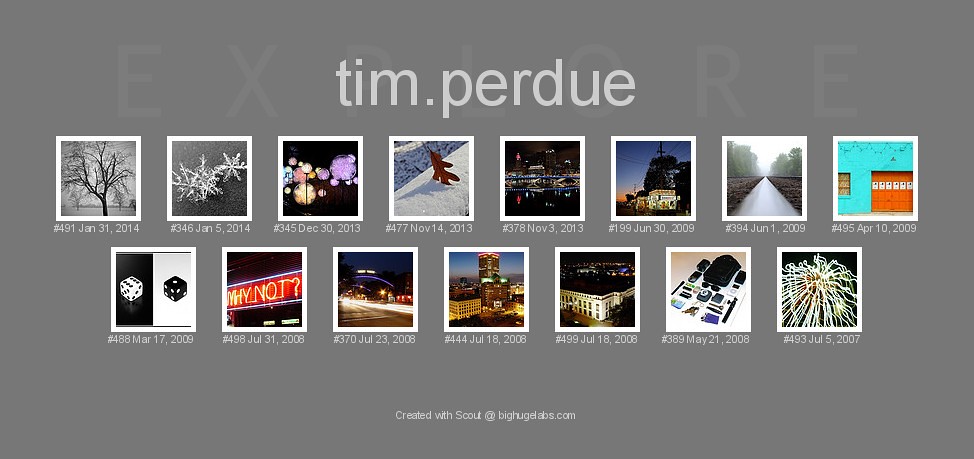The image is a rectangular design, approximately twice as wide as it is tall. The background is flake gray. At the top, faintly written in lighter gray, are the words "explore," and centered over that in lowercase is "tim.purdue." Below this, there are two rows of square photographs, each with a white border and a number and date underneath.

Top Row, Left to Right:
1. A black and white photo of trees, labeled number 491, dated January 31, 2014.
2. A black and white image that appears to be plastic snowflakes, labeled number 346, dated January 5, 2014.
3. A photograph of pastel-colored globes of light in a dark setting, labeled number 345, dated December 30, 2013.
4. A cement background with a rust-colored leaf, labeled number 477, dated November 14, 2013.
5. A nightscape city scene, labeled number 378, dated November 3, 2013.
6. A nighttime image of a lit storefront, labeled number 199, dated June 30, 2009.
7. An image of a waterway or walkway at dusk, labeled number 394, dated June 1, 2009.
8. A turquoise wall with an orange garage door, labeled number 495, dated April 10, 2009.

Bottom Row, Left to Right:
1. A split photograph with white and black backgrounds, featuring black and white dice, labeled number 488, dated March 17, 2009.
2. A neon sign reading "why not?" in yellow and orange, labeled number 498, dated July 31, 2008.
3. A nighttime photo with streetlights or headlights, labeled number 370, dated July 23, 2008.
4. A cityscape at dawn or dusk, labeled number 444, dated July 18, 2008.
5. A white building at night, labeled number 499, dated July 18, 2008.
6. An image of computer or video game components, labeled number 389, dated May 21, 2008.
7. A photo of fireworks, labeled number 493, dated July 5, 2007.

At the very bottom, centered, the text reads: "Created with Scout at bighugelabs.com."